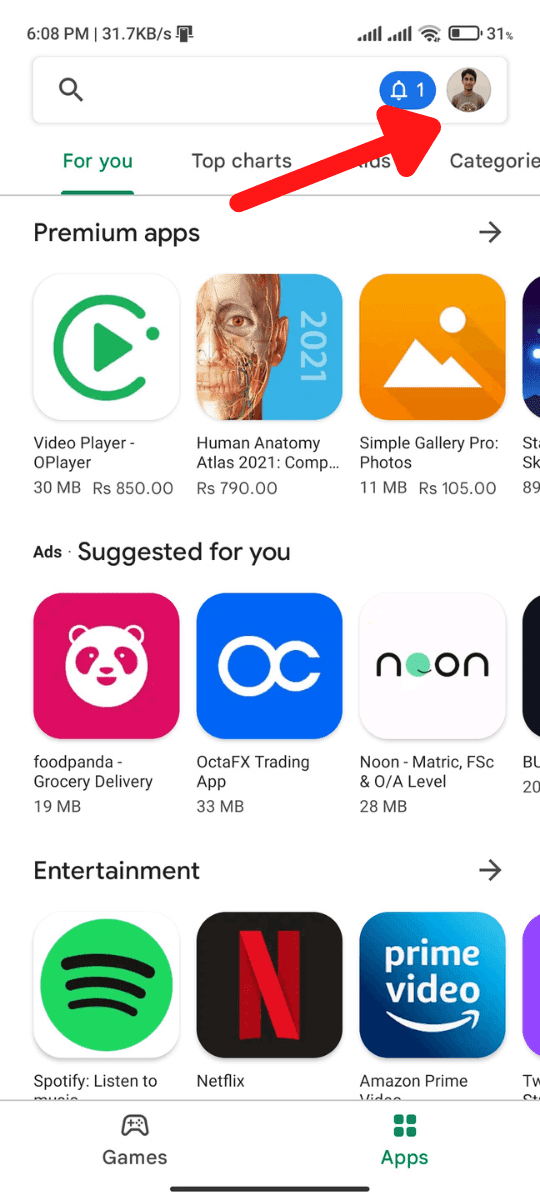The screenshot captures a mobile device interface displaying a variety of apps and system information. At the top left corner, the current time is 6:08 PM. Adjacent to the time, network monitoring speed is indicated at 31.7 kilobytes per second. The top right corner hosts two identical network signal icons. Below this top bar, the home screen is populated with various app icons such as Video Player, Human Anatomy Atlas 2021, Simple Gallery Pro Photos (suggested for you), Food Panda, Grocery Delivery, OctaFX Trading App, Known, Matric, FSC, Amazon Prime Video, Netflix, and Spotify. The colors that dominate the screenshot include vibrant shades of yellow, blue, red, and black, contributing to an aesthetically appealing and organized digital environment.